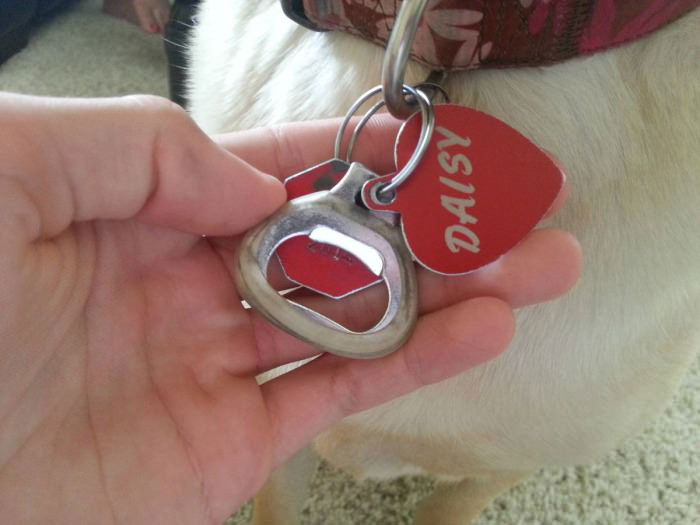In the image, an individual's hand is seen holding the tags from a dog's collar. The focus is on the red heart-shaped dog tag that reads "Daisy" in white letters. This tag is attached to two metal key rings, which also hold a silver bottle opener and another red tag shaped like a stop sign. The dog's collar is a floral design with red, black, and pink colors. Only the dog's chest and front legs are visible, showing white fur with some light tan areas. The background reveals a cream-colored carpet. The scene captures the close-up details of the tags and the person's grip, highlighting the dog's accessories and part of its distinct fur pattern.